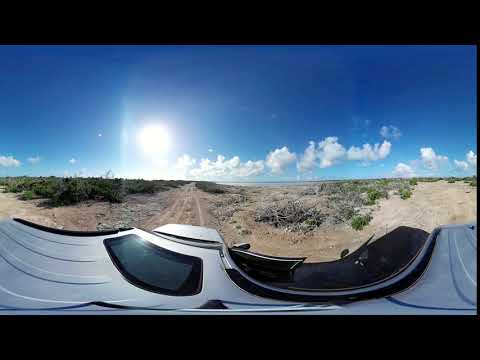The image captures the vantage point from inside a modern, grayish-blue SUV, evident by the visible hood and a part of the sunshade. The SUV is driving down a central dirt road through a vast, open desert-like landscape filled with sand and gravel. To the right, there are distinctive sand dunes with small piles of sand, and dried branches and kindling scattered along the side of the road. On the left, the terrain is more bushy with dark green shrubs. The bright Sun is positioned just above the horizon, illuminating the entire scene with a strong brilliance that accentuates the vibrant blue sky, which transitions from a deep blue above to scattered, fluffy white clouds in the middle. The horizon displays sparse vegetation and possibly a hint of distant water. The overall atmosphere is bright and somewhat arid, reinforcing the desertlike feel of the landscape.